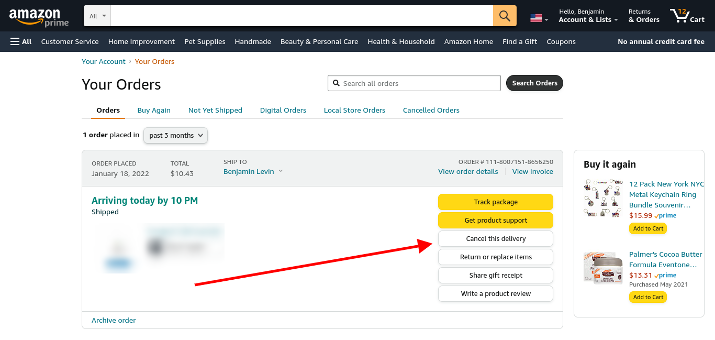The image is a screenshot taken from an individual's Amazon webpage. At the top, the dark Amazon Prime header is visible, featuring a search bar, an American flag icon, and a welcome message stating "Hello, Benjamin." The navigation options "Accounts & Lists," "Returns & Orders," and a cart icon indicating 12 items are also present in this section.

Central to the image, a red arrow is placed conspicuously, pointing from an area near where a product image would typically be displayed. This arrow extends across the screen to highlight the "Cancel this delivery" option. Additionally, above this option, there are links for "Track package" and "Get product support."

Further down, the screenshot shows that the order was placed on January 18, 2022, with a total of $10.43, and is addressed to Benjamin Levin. Despite efforts to cancel, the order status indicates it is "arriving today by 10 p.m." and has already been shipped, implying that cancelling might not be successful, and the item might need to be returned upon delivery.